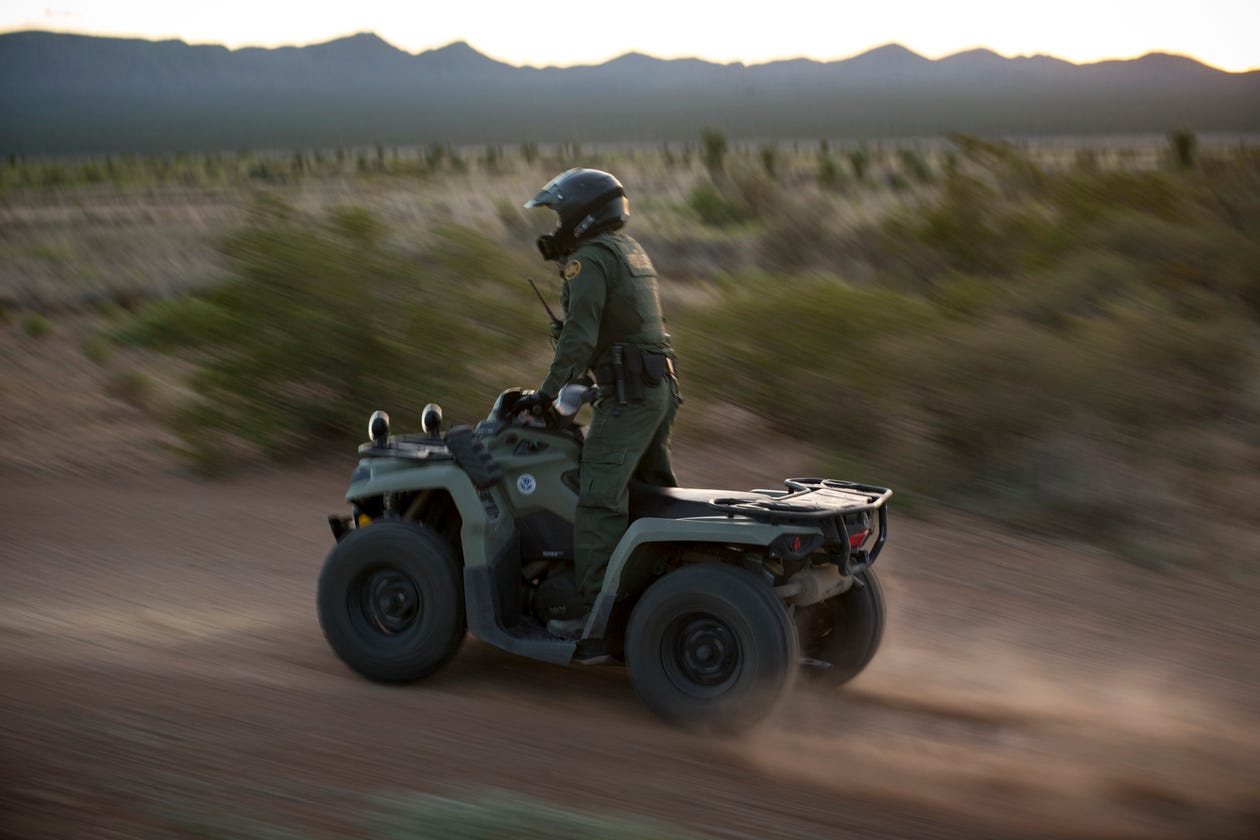The image captures a dynamic scene of a man riding a four-wheeled ATV through a dusty desert landscape. The focus is sharply on the rider, who drives standing upright, his green uniform accented with yellow badging and a black helmet making him noticeable. The ATV, with its dark green body and black rubber tires, appears to be barreling down a sandy path, kicking up dust in its wake. In his hand, the rider clutches a walkie-talkie, hinting at a role that necessitates swift communication, possibly for a Border Patrol or similar duty. Above, the sky hints at an early sunrise, casting a bright yellow glow that outlines the shadowed mountain range in the background. Though blurred, the surroundings feature sporadic bushes and rugged terrain, enhancing the sense of speed and movement in this vivid outdoor adventure.